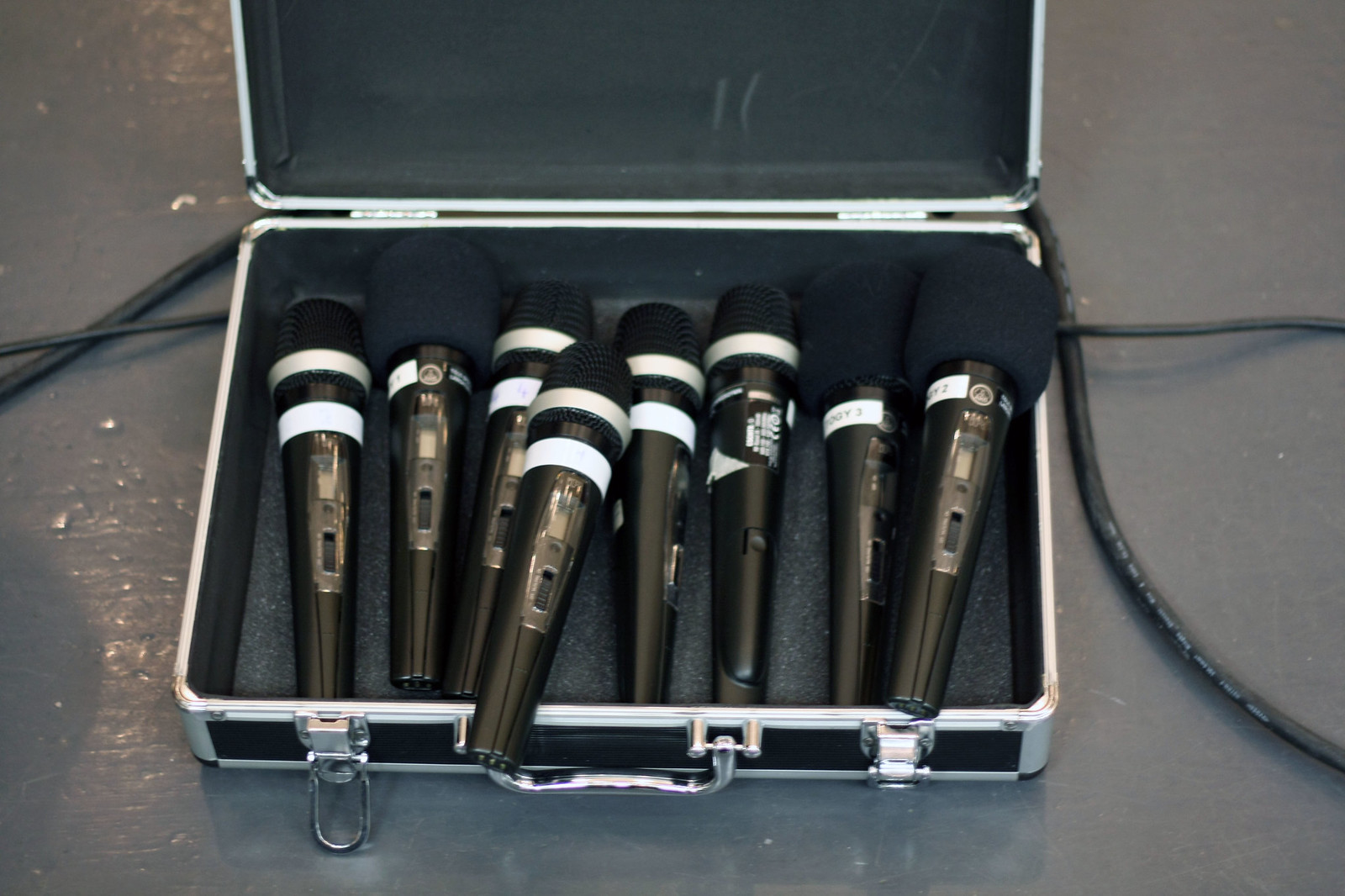The image depicts a black and silver carrying case, open and padded inside, positioned on a gray painted concrete floor. The case contains eight black microphones, each with white stripes: five have two white stripes, while three have one white stripe and feature a foam cover over the mouthpiece. The microphones are neatly arranged in the case, though two of them are slightly sticking out. Surrounding the case, there are several cables—some thick and some thin—running left to right, suggesting preparations for a musical event. The case is equipped with two traditional latches and a handle, indicating it is designed for secure transport yet lacks any keyholes.